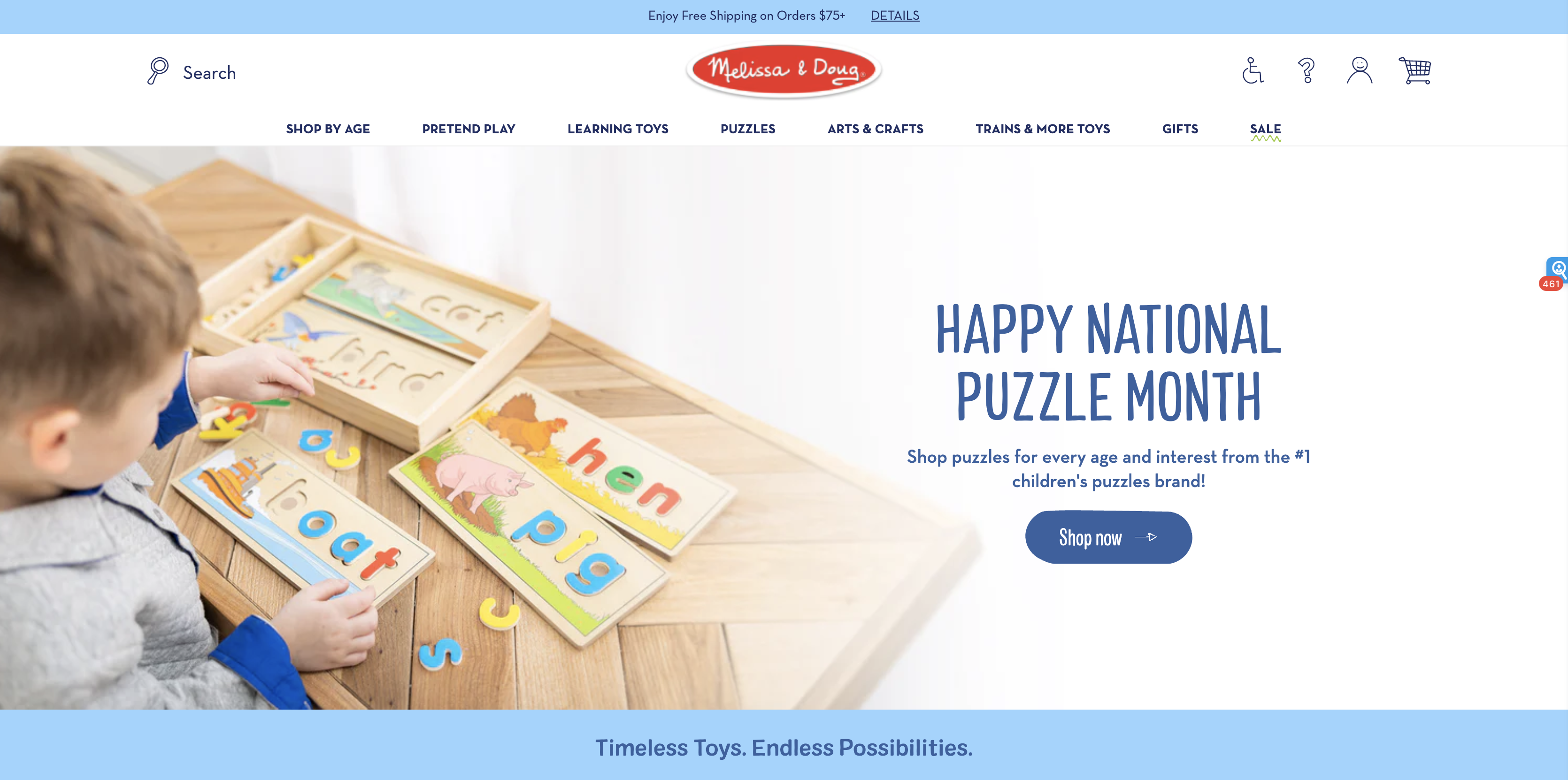### Detailed Caption

This image is a screenshot from the Melissa and Doug website, showcasing various features of the homepage. 

#### Header Section:
- **Top Bar:** A light blue horizontal bar spans the top of the page. In dark blue text, it reads, "Enjoy free shipping on orders," followed by a small, unclear number. To the right, there is a "Details" link.
  
- **Main Header:** Below this bar is the main navigation header. 
  - **Logo:** Centered in this section is the Melissa and Doug logo. It is an oval-shaped, red emblem with "Melissa and Doug" written in white cursive letters, bordered with a drop shadow.
  - **Icons:** To the far left is a search button. On the right side, various icons are displayed: a wheelchair icon for accessibility, a question mark for help or FAQ, a user icon for account access, and a shopping cart icon.
  - **Navigation Menu:** The central navigation menu is listed horizontally in dark blue capital letters. The categories include: 
    - Shop by Age
    - Pretend Play
    - Learning Toys
    - Puzzles
    - Arts & Crafts
    - Trains & More Toys
    - Gifts
    - Sale

#### Hero Section:
- **Primary Image:** Below the navigation menu is the hero section, featuring a large image of a young boy playing at a children’s table. He is interacting with wide cards that depict various objects and animals alongside their corresponding names. Visible cards include a hen labeled "HEN," a pig labeled "PIG," and a boat labeled "BOAT."
  
- **Promotional Text:** To the right of the image, which fades to white, promotional text in large blue capital letters reads, "Happy National Puzzle Month." Below this is smaller subtext promoting the puzzles: "Shop puzzles for every age, interest from the number one children’s puzzle brand." 

- **Call to Action:** There is a "Shop Now" button beneath the promotional text. This button is blue with rounded edges and features white text and an arrow.

#### Footer Section:
- **Tagline:** The section is concluded with another light blue bar stretching across the image. Centered within this bar, in dark blue text, it reads, "Timeless Toys. Endless Possibilities."

This detailed breakdown encapsulates the various elements present in the screenshot from the Melissa and Doug website.